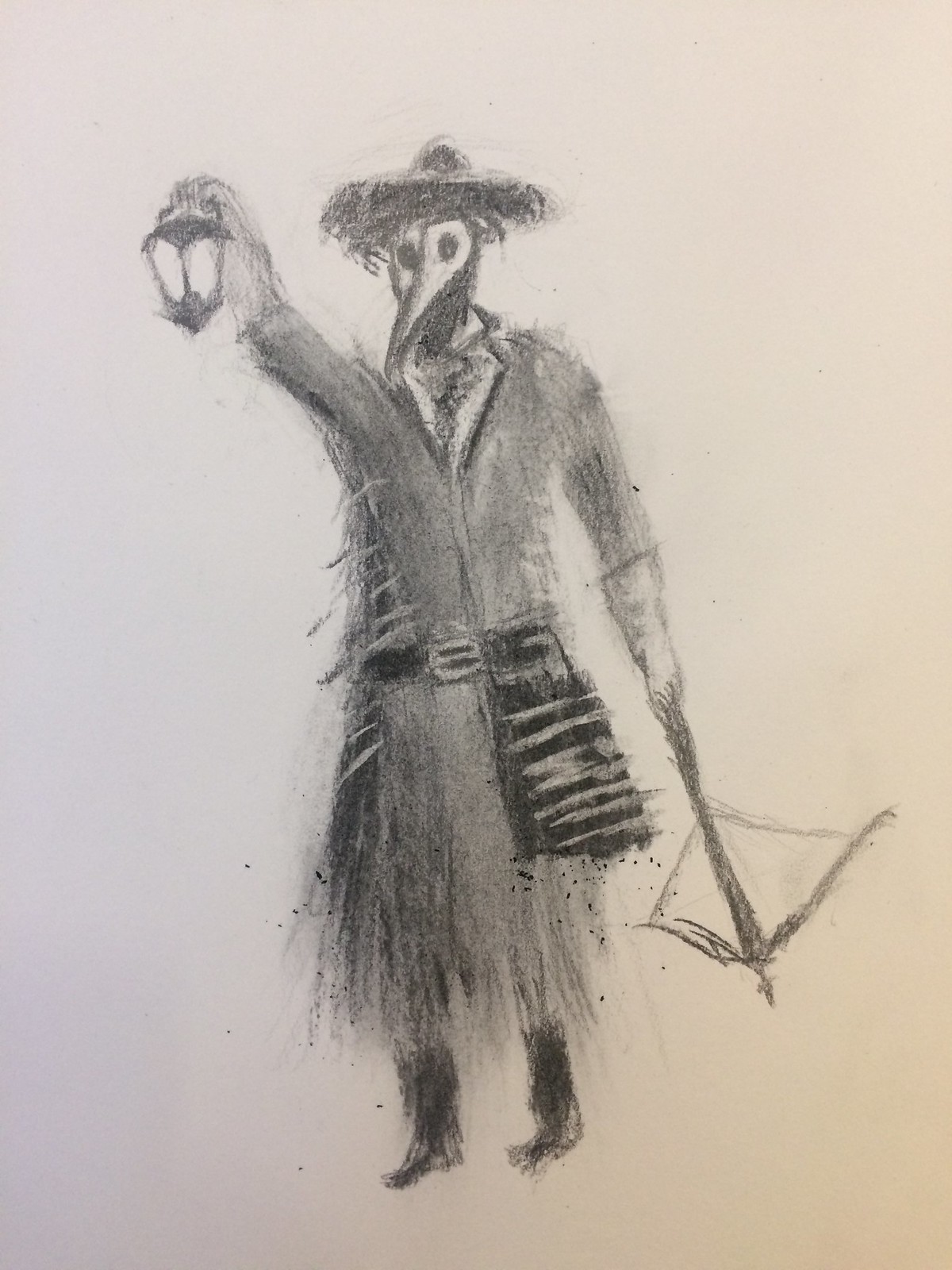The drawing, rendered in vertical alignment possibly with charcoal or graphite, depicts a mysterious figure dressed in a black trench coat that nearly reaches their feet. This figure, which stands against a gradient background transitioning from bluish on the left to pinkish on the right, wears black boots and a large round hat with a pointed tip resembling a sombrero. The figure's face, obscured by a human-like bird mask with dark, piercing eyes and a sharp protruding beak, adds an eerie touch. The figure's right hand holds up a lantern, casting an ominous glow, while the left hand grips a crossbow pointed downward. Additional details include a long fanny pack or bag attached to the figure's belt, accentuating the character’s enigmatic and somewhat menacing appearance.